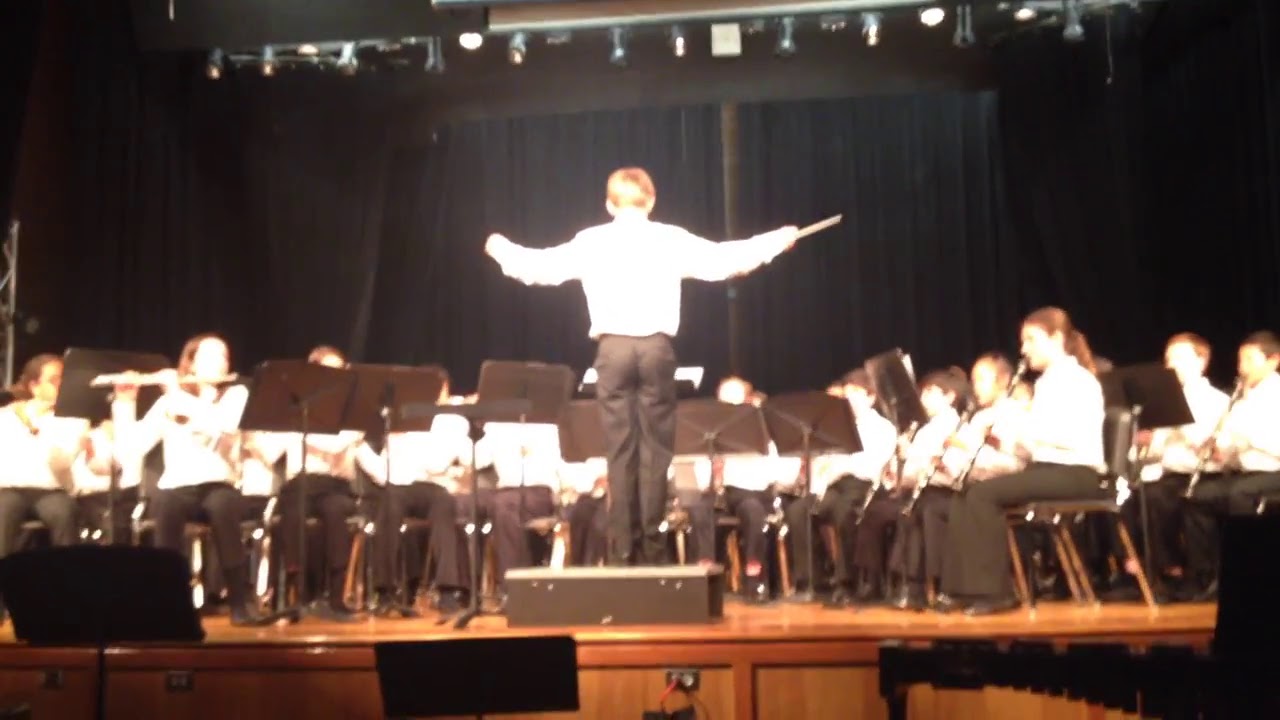In the photograph, taken from the audience, a child conductor is orchestrating a band on a light brown wooden stage. The conductor, dressed in a long-sleeved white shirt and black pants, stands on a small black pedestal to ensure visibility for both himself and the musicians he’s directing. He has blonde hair and his back is to the camera, with his arms outstretched in mid-conduct. The backdrop is a prominent black curtain, and stage lights above cast an ambient glow, affecting the image quality and slightly washing out facial details.

The ensemble consists of approximately 30 to 40 musicians, all dressed uniformly in black bottoms and white tops. In the front row, flute and clarinet players are noticeable. The first chair flute players are positioned on the left side and are observed sharing sheet music, while the first chair clarinet players are on the right side with the last row consisting of more clarinet players. Additional musicians holding various instruments can be seen seated behind them, with music stands and holders set up in front of each player. The photograph has no text or date markings.